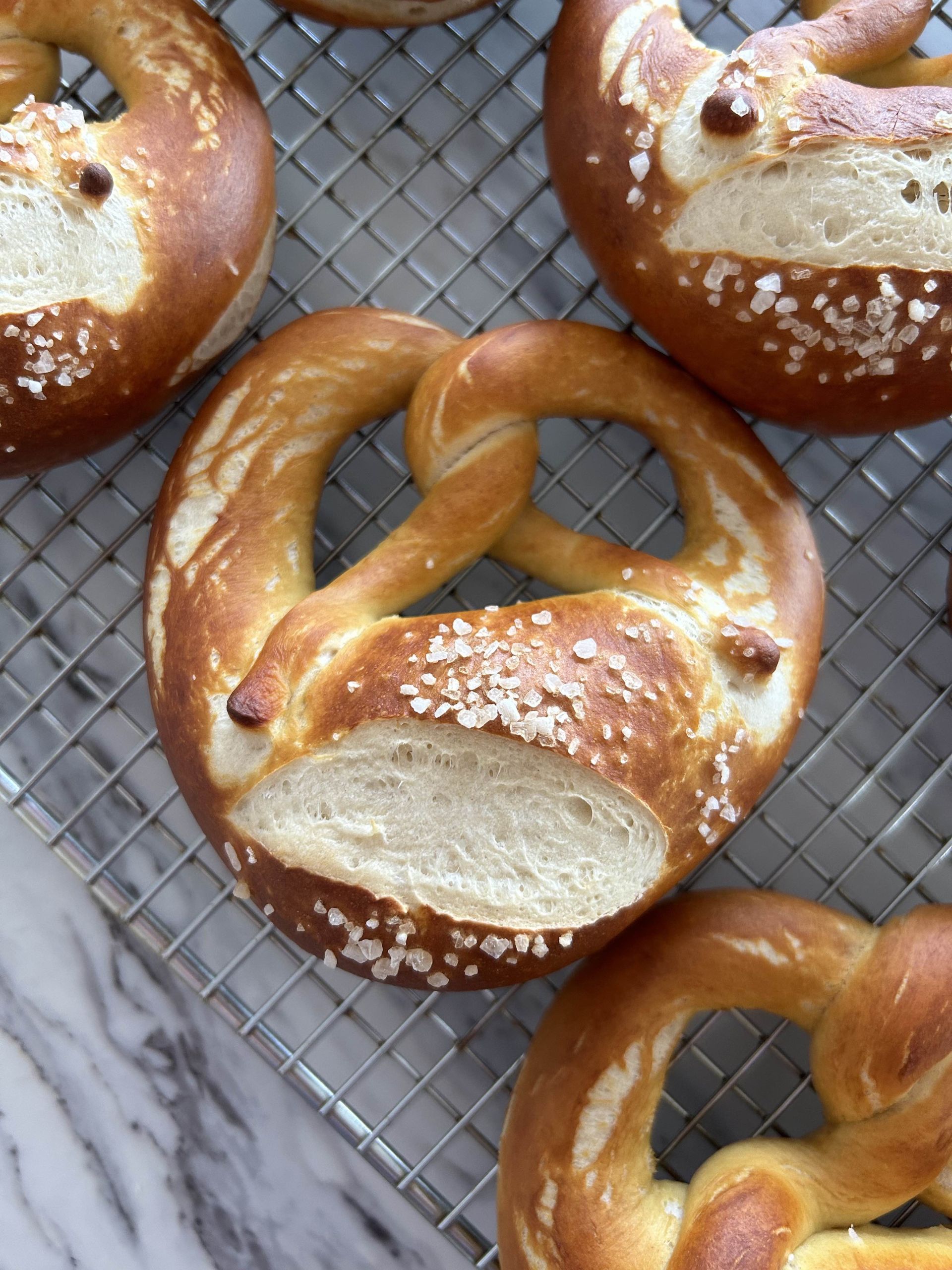The image shows a cooling rack with four homemade soft pretzels resting on it. The pretzels appear to be imperfectly shaped, with areas that are thicker or thinner than others. The central pretzel is fully visible and has a sizable piece missing from its bottom portion, suggesting it was sliced off. The pretzels are sprinkled with salt, though not uniformly; most of the salt is concentrated towards the bottom sections, with the loops largely lacking salt. Some of the pretzels, including one in the top right corner, show signs of being slightly burnt. The cooling rack, a metal mesh type, is placed on a white marble surface featuring gray and black veining. A small portion of a fifth pretzel is just visible at the top of the image.